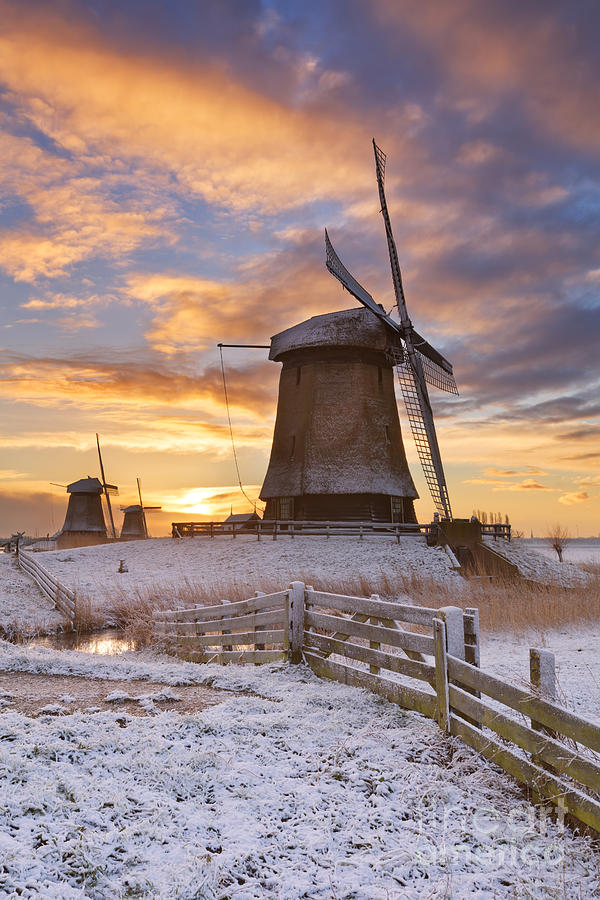A picturesque scene unfolds at sunset during winter, capturing a windmill prominently in the center. The sky is a canvas of vibrant hues, with the horizon ablaze in orange and yellow and the clouds brushed with shades of blue, creating a mesmerizing backdrop. The windmill, modest in size compared to towering modern turbines, stands atop a small, rustic brown building adorned with black blades. Encircling this structure is a wooden fence that extends into the horizon and fades from view. The snowy grass in the foreground accentuates the serene winter atmosphere. Behind the main windmill, two similar windmills are visible in the distance, adding depth to the landscape. A small pond, surrounded by sparse patches of brown grass and other winter vegetation, adds a final touch of tranquil beauty to the scene.